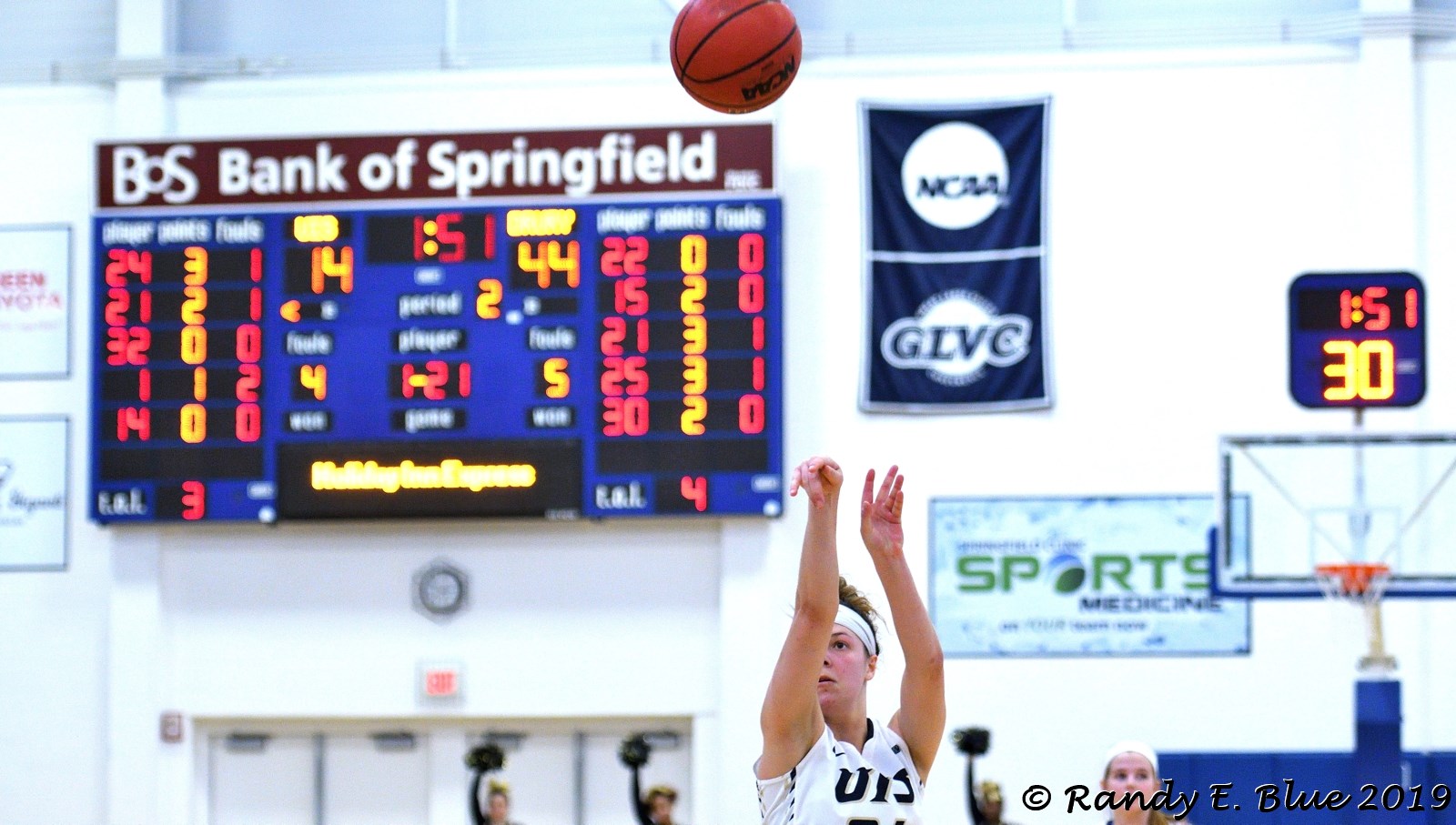In this photograph, a Caucasian female basketball player in a white jersey is captured mid-action, making a free throw. Her arms are lifted straight as the basketball soars through the air. The setting is a large basketball gymnasium with a white wall and white exit doors. Prominently displayed in the background is a scoreboard featuring the text "BS Bank of Springfield" in blue with red lettering, showing a score of 44-14. Above the hoop behind her is a 32nd shot clock. The scene also includes an NCAA banner and a sign for sports medicine. Three cheerleaders with black pom-poms are visible against the white wall. Another female basketball player stands directly behind the shooter. The photograph, credited to Randy E. Blue from 2019, bears his name and a copyright symbol in the far-right corner.